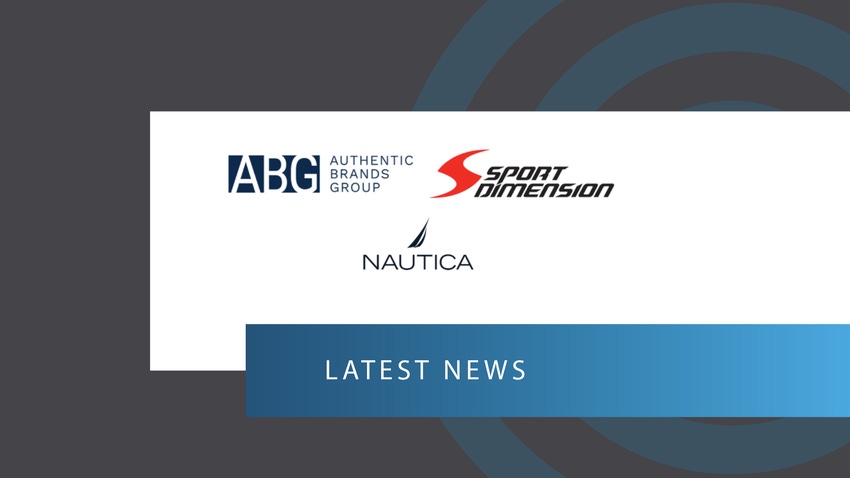This image is a horizontally oriented, digital poster featuring Graphic Design Typography elements. The background is dark gray accented by a dark aqua circle motif on the right. Central in the composition is a large white horizontal rectangle bordered by a dark blue outer rectangle, creating a cohesive frame. Below the white rectangle, a lighter blue horizontal stripe extends, with white text reading "Latest News."

Inside the white rectangle, at the top left, is a black logo featuring the white letters "A, B, G," representing Authentic Brands Group, whose name is written in black text aligned to the left. Adjacent to this is a red swash-shaped "S" logo, next to the black italicized text "Sport Dimension." Below these logos, towards the bottom, sits the Nautica logo— a simple dark sail design above the word "Nautica."

To the right side of the image, the white rectangle and the lighter blue stripe align perfectly with the dark blue border, which comprises two circles—one white and the other a lighter blue—forming a partial outline that does not interrupt the white or lighter blue sections. The overall layout emphasizes a clean, organized structure with a focus on clarity and brand recognition.